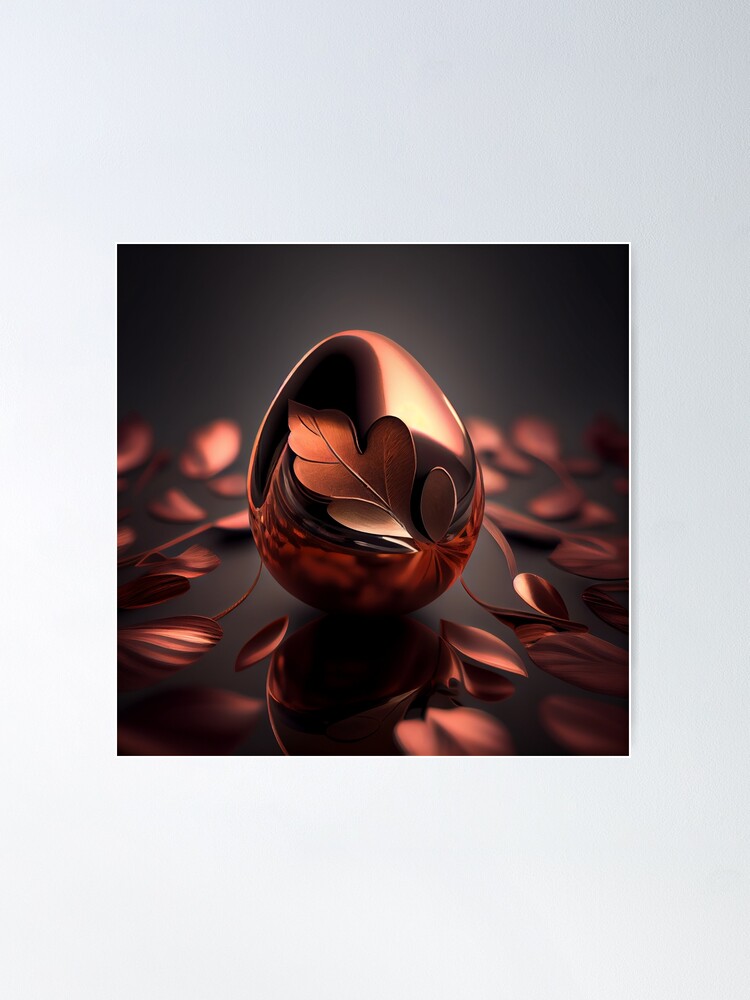The image portrays a high-quality, photorealistic render set against a black and blackish-gray background. Central to the composition is an egg-shaped decorative object, crafted from a bronzy, sun-setting afternoon hue with a touch of rose gold, giving it an orangish-bronze appearance. Adorning this metallic egg is a textured leaf, designed to appear as though it is naturally peeling off the surface. The leaf showcases intricate vein details in a lighter tone. Surrounding the egg, scattered across a black, reflective, and matte-finish surface, are numerous out-of-focus, textured bronze metal leaves and petals. These elements frame the central egg, further enhancing the thematic consistency and offering a modern, new-age aesthetic to the photograph.